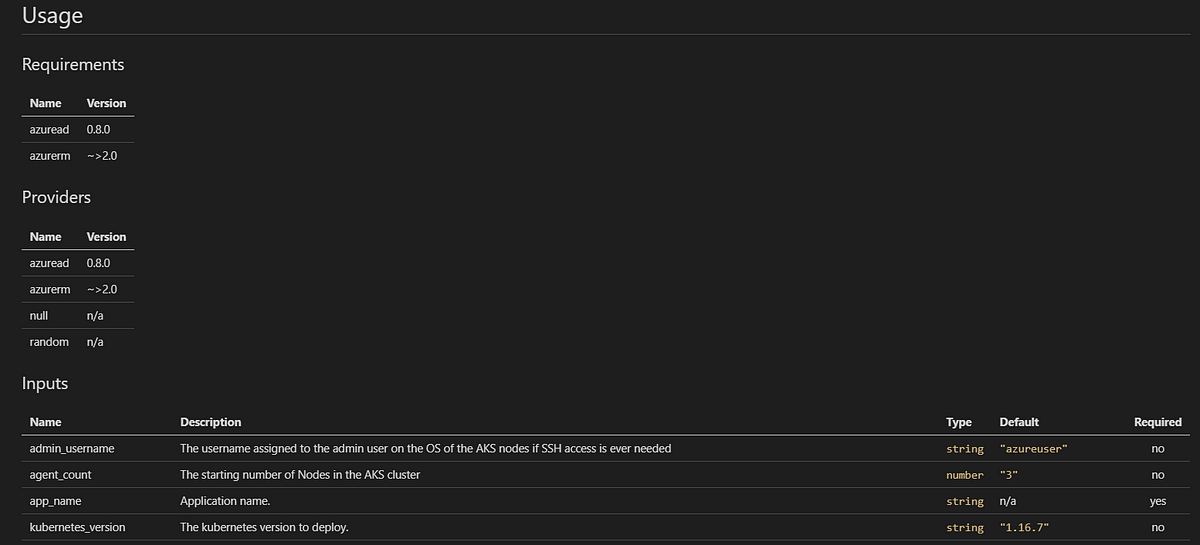The image displays a usage screen for a complete computer system, characterized by its all-black background with white text. The layout of the text is concentrated on the left-hand side and bottom of the screen, leaving a large, unoccupied black area in the middle. 

In the top-left corner, the word "Usage" is prominently displayed in white font. Directly below it, a white horizontal line spans the width of the screen. Following this division, the next section is labeled "Requirements," under which there are two subcategories: "Name" and "Version," providing specific details about the computer system.

The subsequent section is titled "Providers," which lists four providers, each accompanied by its corresponding name and version details. 

Finally, the bottom section is labeled "Inputs," presented in a chart format with multiple categories: "Name," "Description," "Type," "Default," and "Required." This section enumerates various programs that are utilized within the system, each classified under these headings.